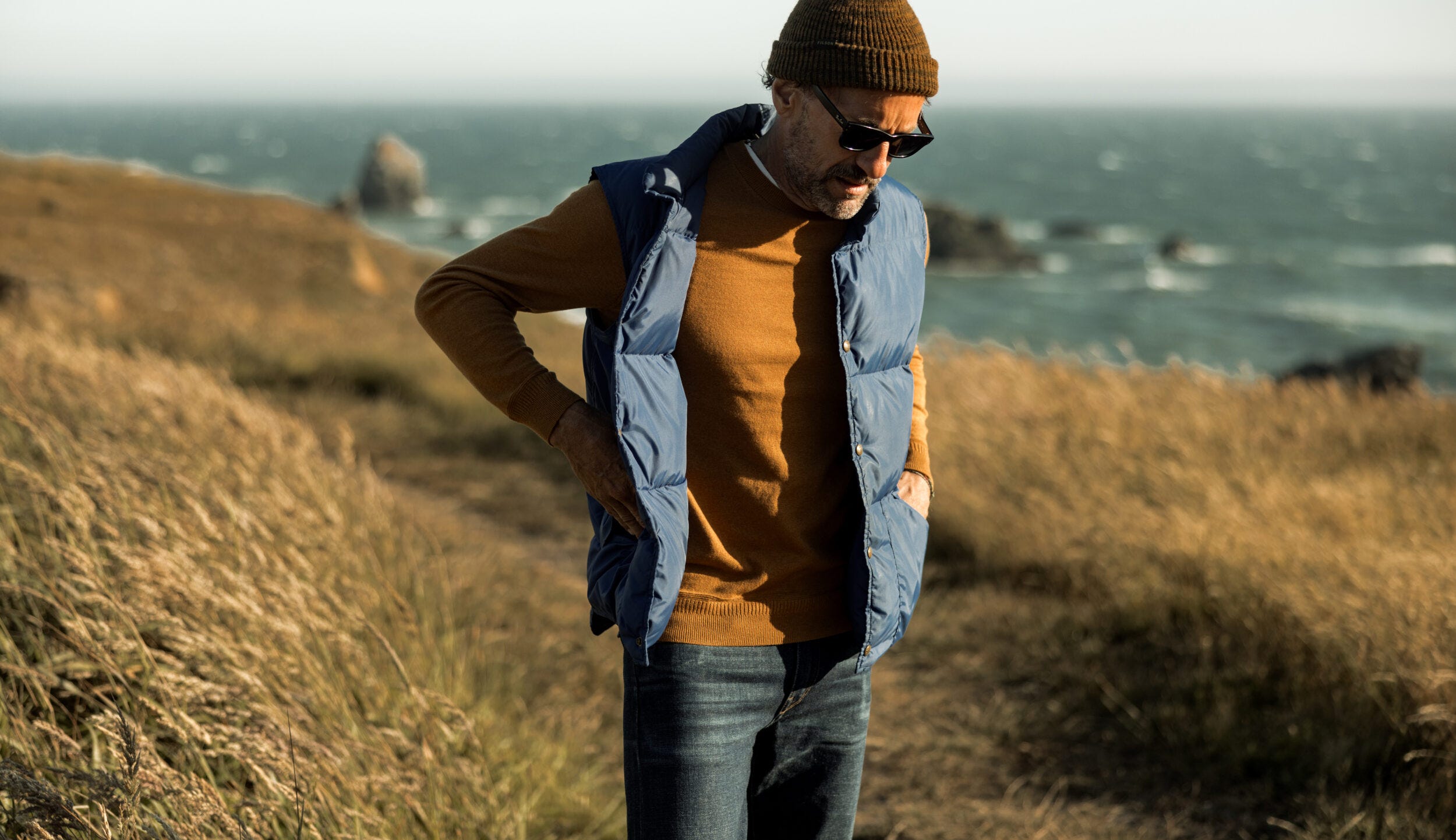The image depicts a middle-aged Caucasian man, likely in his mid-40s to early 50s, standing on a rough path surrounded by tall, brown grass, about two feet high, which sways like wheat. The setting suggests a fall or winter day, with a hazy, gray skyline adding to the somber atmosphere. The man is dressed in a tan sweater layered under a blue, sleeveless puffer vest, and wears denim jeans. He accessorizes with a brown knit beanie, black sunglasses, and has a bit of scruff for a beard and goatee. His left hand is tucked into his vest pocket while his right hand rests against his side. He appears to be looking down contemplatively, with a slightly sad demeanor. Behind him, the landscape opens up to a choppy ocean with large boulders emerging from the water, further enhancing the rugged beachside cliff setting.